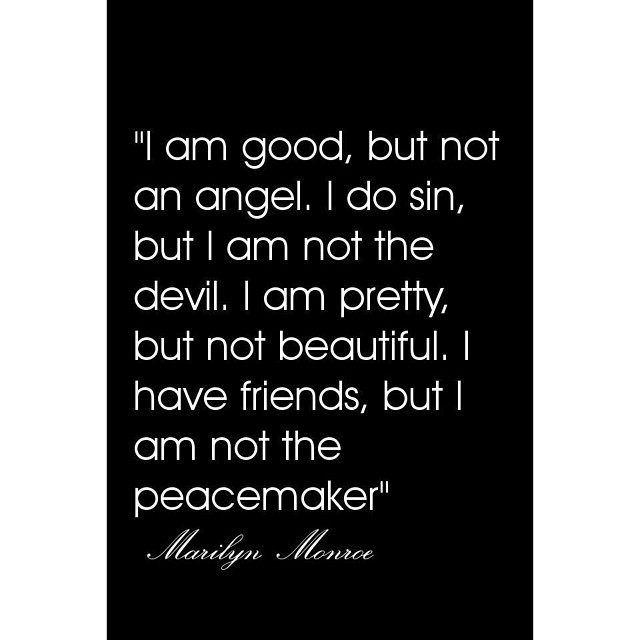The image is a vertically-oriented rectangular poster with a solid black background. It features a quote in white text, written in a playful, somewhat juvenile font resembling Comic Sans. The quote is formatted line by line and centered on the black background. It reads: 

"I am good, but not an angel. I do sin, but I am not the devil. I am pretty, but not beautiful. I have friends, but I am not the peacemaker."

The text spans nearly the full width of the poster with slight margins on the top and bottom. The quote is attributed to Marilyn Monroe, whose name appears at the bottom of the poster in a smaller, elegant cursive script, angled to the right. The inscription aligns neatly along the bottom center of the image, providing a contrasting sophistication to the primary text. The overall design is reminiscent of a decorative mall gift shop poster, with a timeless yet modern appeal.